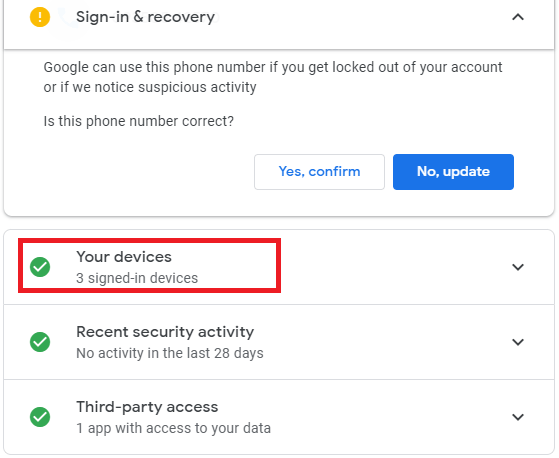In this screenshot of a webpage, several rectangular boxes are outlined in light gray with a white background. In the upper left-hand corner of the image, there's a bright yellow circle containing a white exclamation point. Adjacent to the circle is black text that reads "Sign-in & Recovery." On the far right-hand side of this same box, there is a black arrow pointing upward. Below this, black text reads: "Google can use this phone number if you get locked out of your account or if we notice suspicious activity. Use this phone number correct."

Below this message are two rectangular-shaped buttons. The first button is white, outlined in gray, with blue text that reads "Yes, confirm." The second button is bright blue with white text that reads "No, update."

Below these buttons are three rectangular tabs, each featuring a green circle on the left-hand side with a white check mark in the center. Each tab has a black text heading. The first tab reads "Your devices," followed by "3 signed-in devices" in gray text. The second line reads "Recent security activity," followed by "No activity in the last 28 days" in gray text. The third line reads "Third-party access," followed by "One app with access to your data" in gray text.

The first tab, labeled "Your devices," is outlined in a thick, bright red border, which encompasses the green circle with the white check mark, the "Your devices" text, and the "3 signed-in devices" text in gray. At the end of each of these tabs, there is a black arrow pointing downward on the right-hand side.